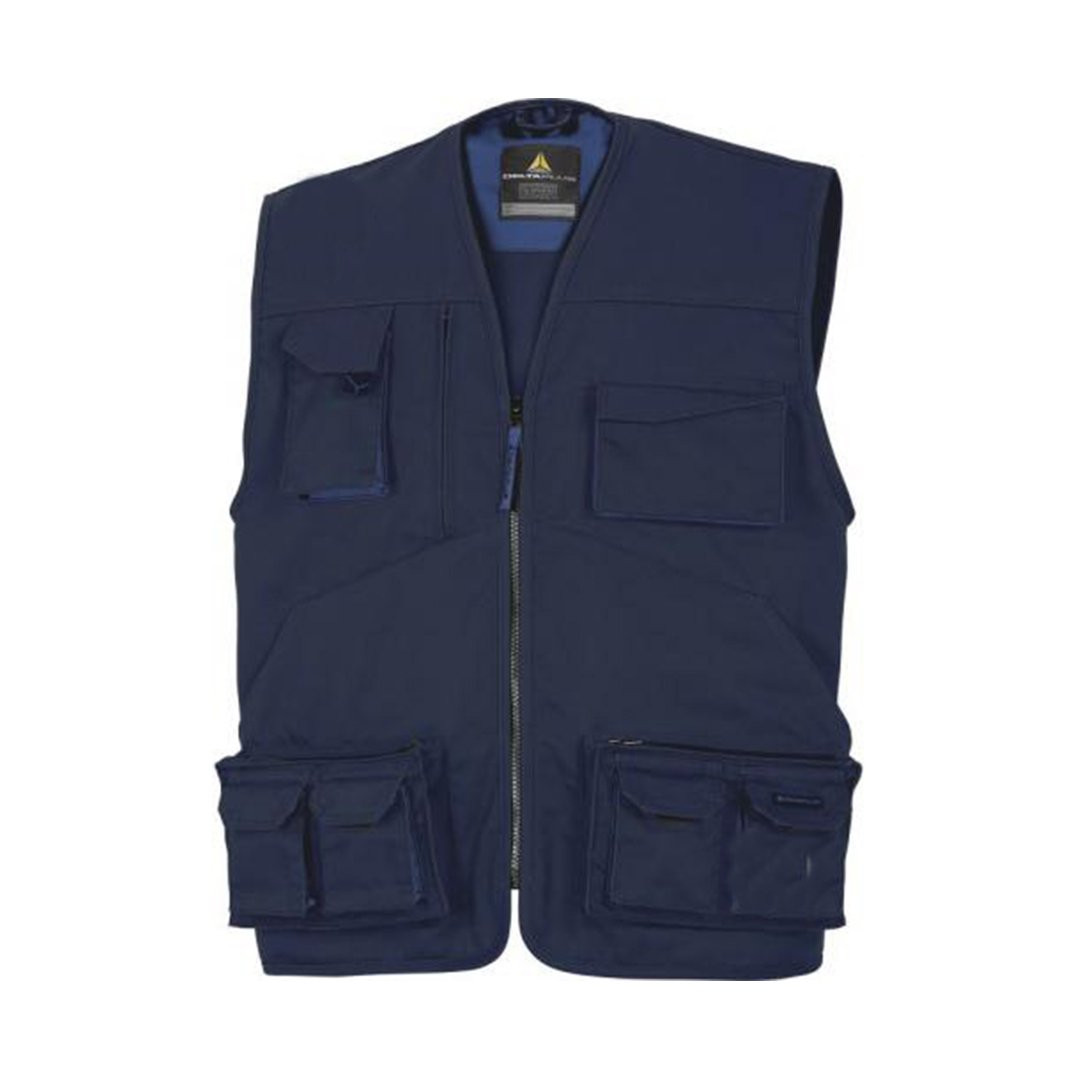This is a vertical image of a dark blue, almost navy blue, outerwear vest, set against a solid white background. The vest, adorned with numerous pockets, is designed for activities such as sports, hunting, and fishing. It features a v-neck opening without a collar and a front silver zipper, which is currently zipped up about two-thirds of the way. On the inside back of the vest, a black label is visible against a lighter blue interior, indicating the manufacturer and washing instructions, though the text is blurry and unreadable.

The vest is equipped with a total of six pockets on the front. At chest level, the right side has a horizontally rectangular pocket, while the left side features a vertically rectangular pocket with a flap closure. The lower part of the vest showcases double-pocketed sections on each side. Each section includes a larger pocket with a zippered component behind two vertically aligned flap-closure pockets. Additionally, there are single pockets on each side of the vest, also covered by flaps, and a strap is present at the back of the collar. The thoughtful design of these pockets and closures suggests they are secured by Velcro to prevent items from falling out.